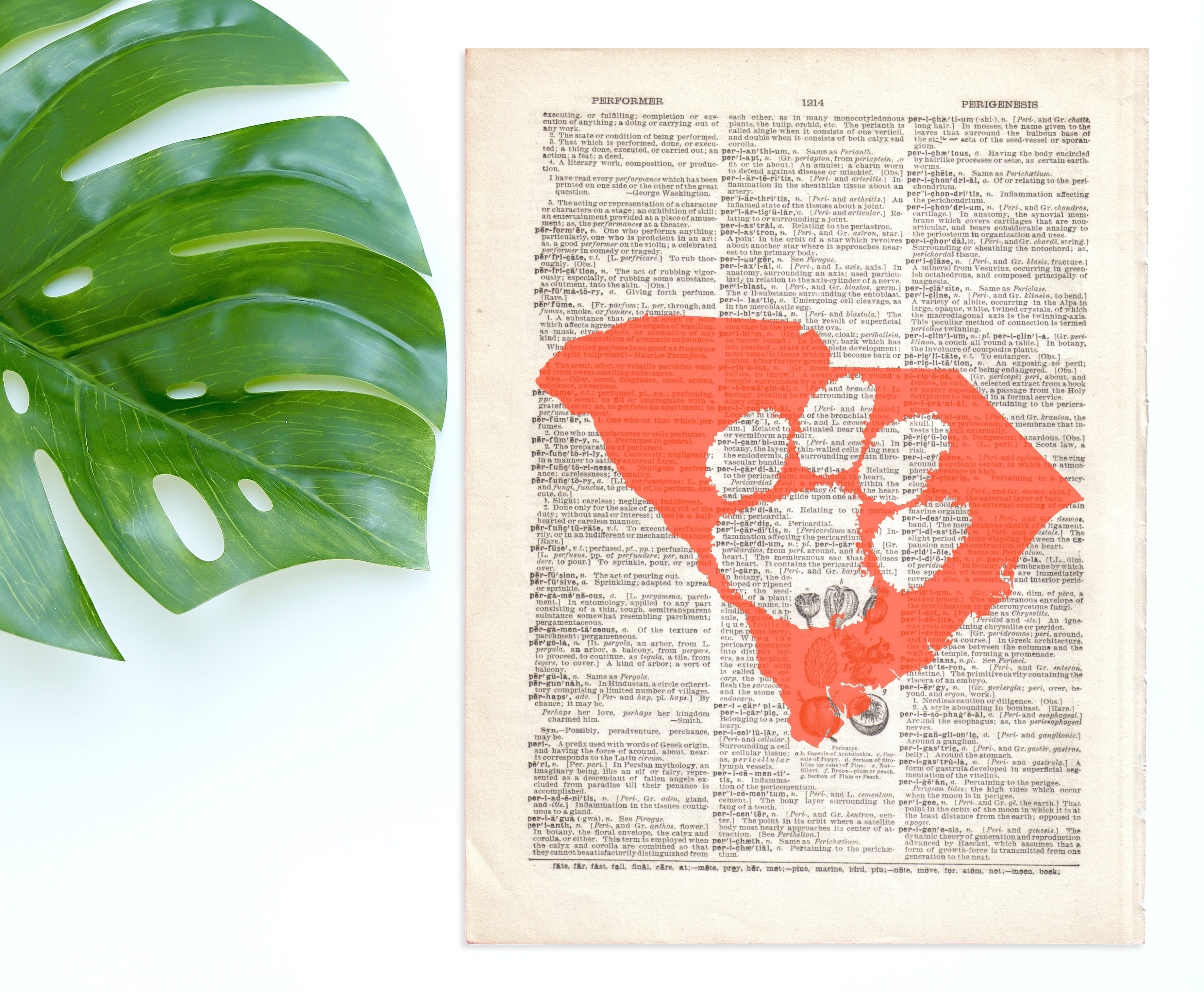The image depicts a page seemingly torn from a dictionary or encyclopedia, displaying three neatly organized columns of words, each with bolded entries followed by definitions. At the top of the left column, the header reads "PERFORMER," the middle column is labeled "1214," and the right column features "Ferio and Este." Overlaid on this text is a splash of abstract orange paint resembling the shape of South Carolina, within which a paw print—potentially representative of the Clemson Tigers logo—reveals the underlying words. Flanking the torn page to the left is a large, perforated green palm leaf. The paper rests against a white backdrop, blending elements of text, illustration, and nature in a visually striking composition.